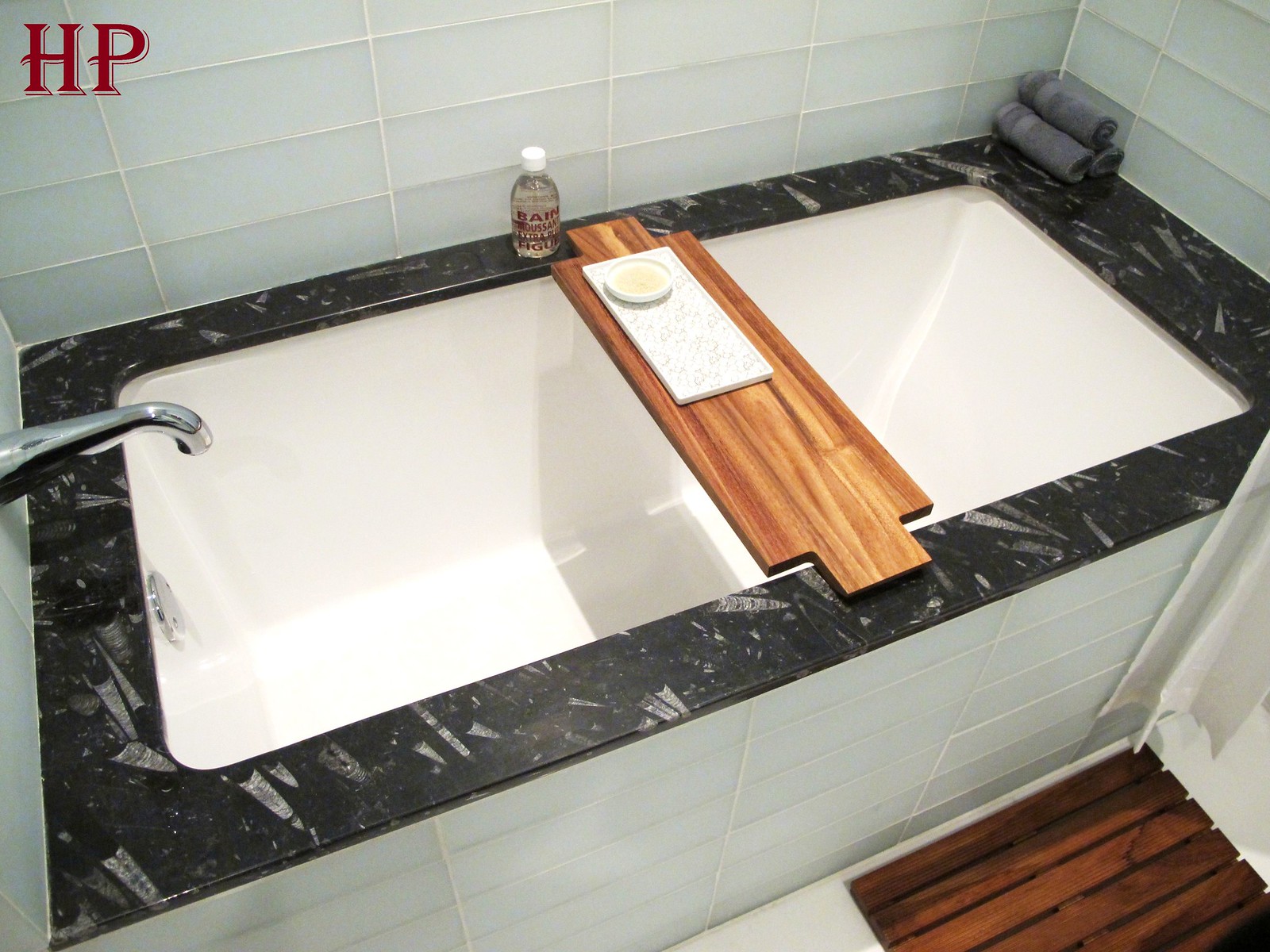The image captures a luxurious bathtub setting with meticulous detailing. In the top left corner, there is a red watermark labeled "HP". The wall behind the tub is adorned with wide, rectangular white tiles, with the grout color almost matching the tiles. The floor features similarly white tiles, which appear broader. A medium-dark brown wooden teak bath mat is placed on the floor, adding a natural element to the scene.

The front of the bathtub is tiled with the same white rectangular tiles as the wall, creating a seamless look. Contrastingly, the top edges of the bathtub are made of black marble with elegant white streaks. Inside the bathtub, in the back right corner, there are three neatly rolled blue-gray towels, contributing to the spa-like atmosphere. The tub's silver spout is noticeable, although the controls for turning on the water are not visible. The bathtub itself is white and seems compact, suggesting it is suitable for a smaller-sized adult.

Spanning across the bathtub is a wooden tray, stylishly placed for convenience, likely intended for reading, drinking, or dining while bathing. On this wooden tray, there is an indeterminate whitish block and a small circular object, the purposes of which are unclear. Additionally, a bottle of soap is placed nearby on the tray, adding to the functional yet elegant aesthetic. The overall setting exudes an upper-class vibe, emphasizing comfort and sophistication without being overly opulent.